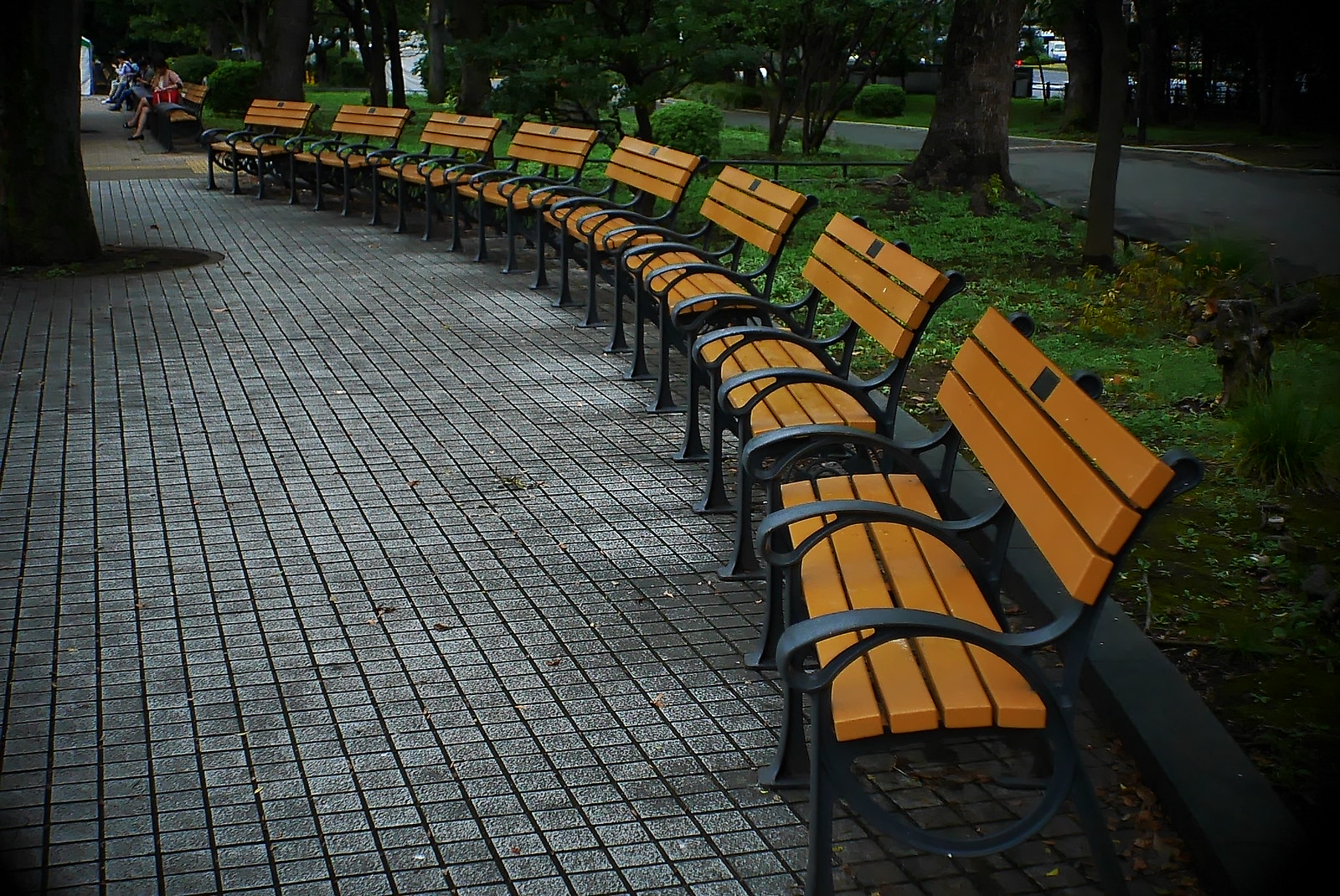A series of approximately eight identical park benches are arranged in a semi-circle in a well-shaded park area. Each bench features black wrought iron sides, three black armrests, and an orange-burnt hue on its wooden seat and backrest panels. The benches also have a small, black square tag at the top center, potentially serving as a dedication plaque or manufacturer’s mark. The ground in front of the benches consists of neatly arranged stone tiles, each forming small squares. Behind the benches, green foliage including trees, bushes, and hedges provides a natural backdrop. In the distance, people can be seen sitting on benches, with one woman wearing a pink jacket and holding a red bag. A large tree on the right side is surrounded by a circular mulch area, indicating park maintenance. Beyond the park, a street and nearby housing peek through the branches, adding to the urban setting.